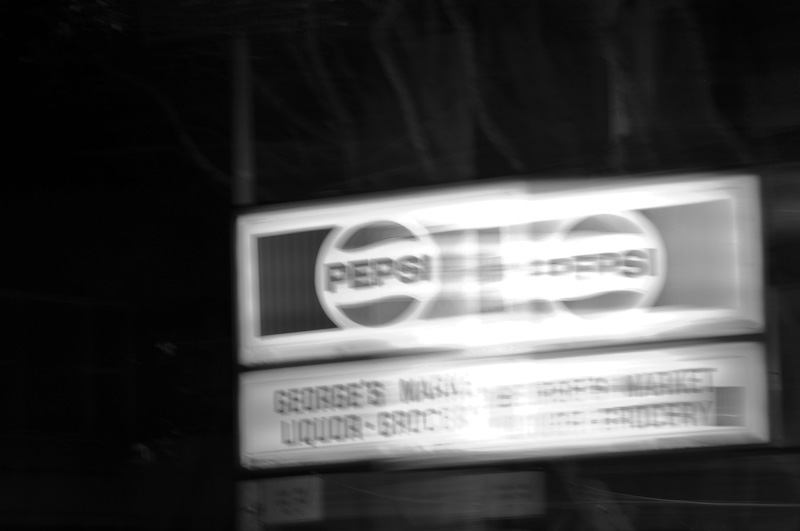The image is a blurry, black-and-white photograph, likely taken at night, outdoors. The focal point of the image is a set of illuminated signs. At the top, there are two side-by-side Pepsi logos on a long rectangular sign. Below the Pepsi sign, there is another rectangular sign that reads "George's Market, Liquor, Groceries," although the text is hard to read due to the blurriness. The repetition and overlapping of the signs create a ghosting effect, as if the photo was taken from a moving vehicle. The background is very dark, obscured by blackness with faint outlines of trees. Poles or beams can be seen descending from the top of the image, adding to the outdoor setting. This visual layering and the blur create an abstract, almost surreal composition.